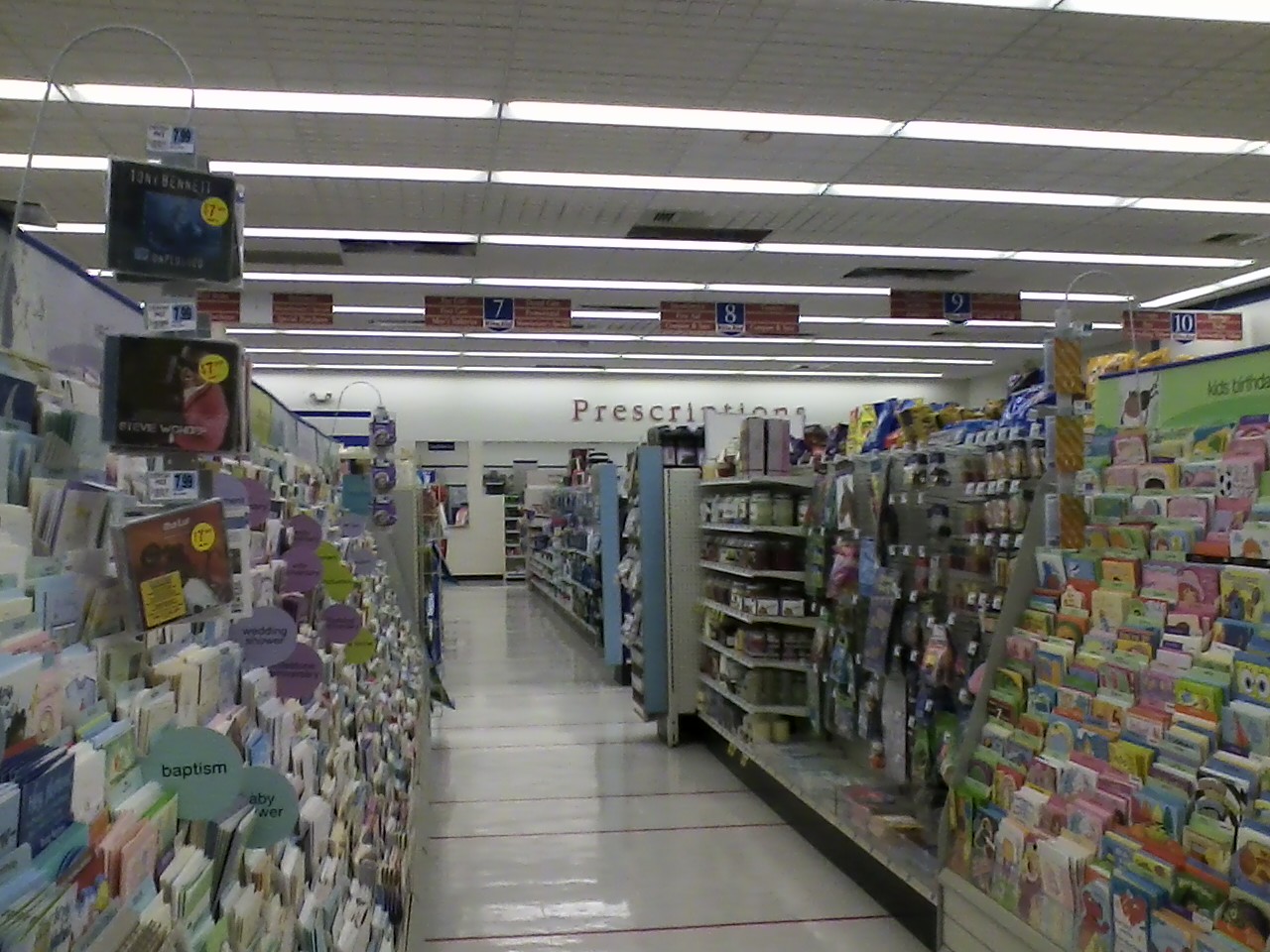This is a detailed photograph of a brightly-lit aisle in a department store or drugstore, captured in a rectangular, landscape orientation. In the background, a prominent sign reads "Prescriptions," indicating the pharmacy section of the store. The aisle is dedicated to greeting cards for various occasions, with an extensive and colorful selection on display. On the left side of the aisle, the cards are arranged by categories such as baptisms and baby showers, while on the right side, a variety of kids' birthday cards can be seen. The aisle shelves and the walls are a clean, uniform white, creating a stark contrast with the diverse and vibrant hues of the greeting cards. The overall composition of the photograph captures the organized, yet lively atmosphere of this section of the store.